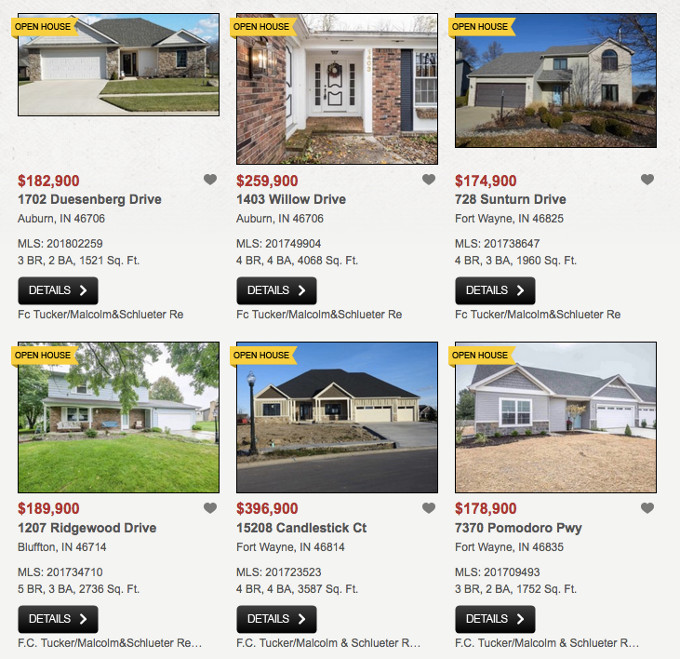The image features six different houses, each marked with a yellow ribbon on the top left corner that reads "Open House." From top left to bottom right, the houses are described as follows:

1. **House 1**: Located at 1702 Duesenberg Drive, Auburn, Indiana, 46706. Listed for $182,900, it offers 3 bedrooms, 2 bathrooms, and spans 1,521 square feet. MLS number is 201802259.

2. **House 2**: Situated at 1403 Willow Drive, Auburn, Indiana, 46706. Priced at $259,900, this property features 4 bedrooms, 4 bathrooms, with a total area of 4,068 square feet. MLS number is 201749904.

3. **House 3**: Found at 728 Sunturn Drive, Fort Wayne, Indiana, 46825. On the market for $174,900, it includes 3 bedrooms, 2 bathrooms, and covers 1,457 square feet. MLS number is 201738647.

(Additional three houses description not provided so assumed only detailed description for these three.)